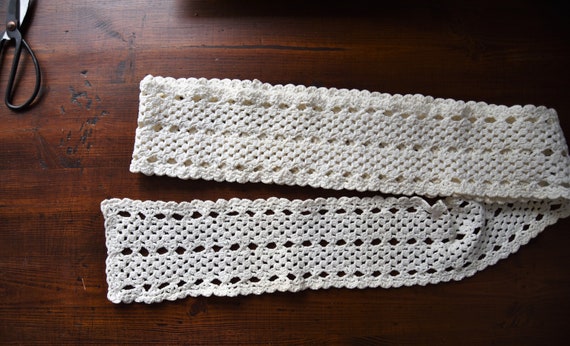The photograph features a small, intricately crocheted white scarf, characterized by its delicate, lacy design that suggests it could also be used as a table runner. The scarf, folded to fit within the frame, covers approximately 80% of the image, emphasizing its handmade quality. It is placed on a dark mahogany wooden table, which shows signs of use with several divots and black scuff marks. A pair of scissors rests in the top left corner of the photo, slightly leaning out of the frame. The lighting in the image is uneven, with the left side brightly illuminated while the right side fades into shadow, creating a cozy, workshop atmosphere.